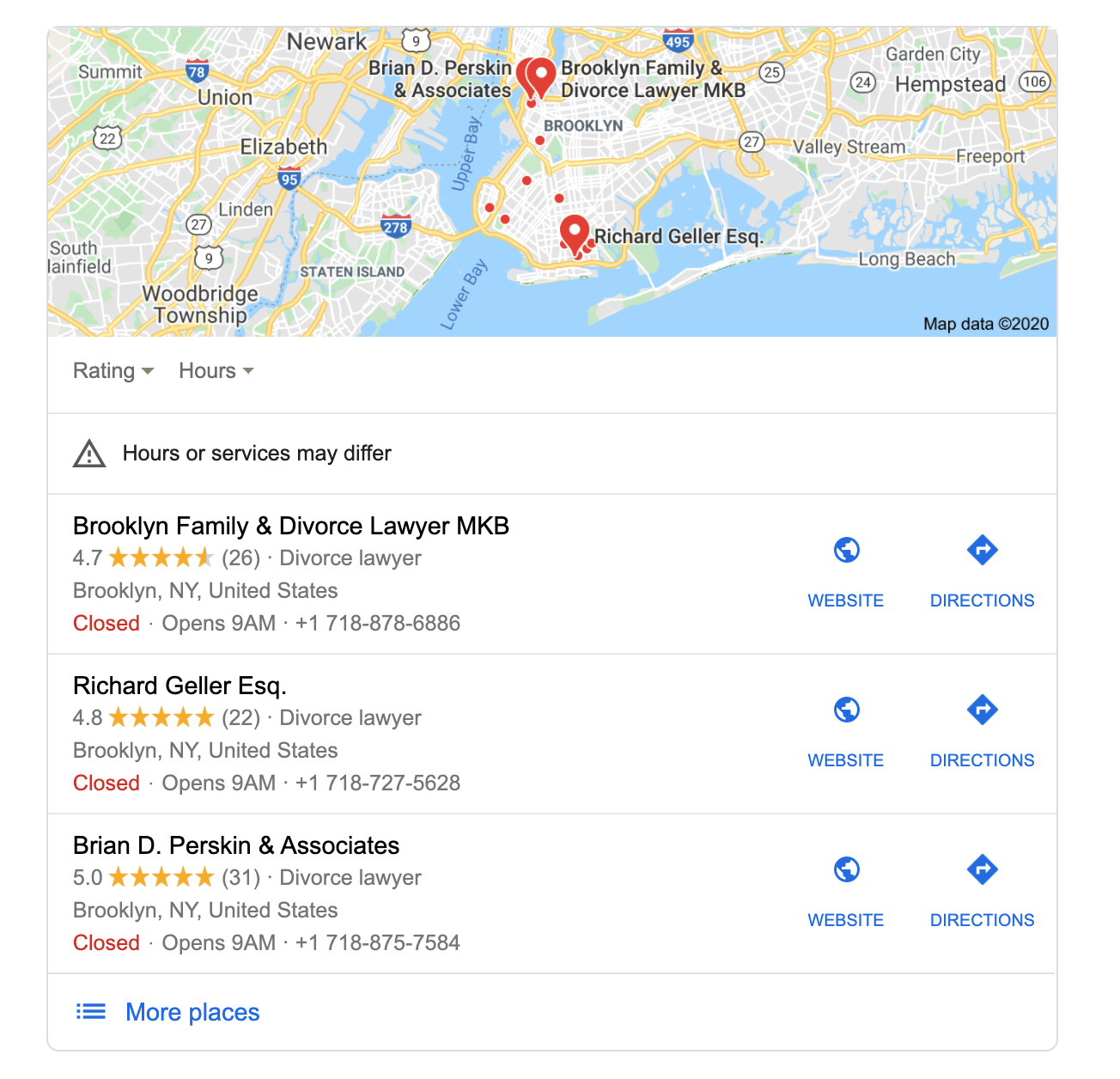The image depicts a user performing a search on Google Maps. The top third of the screen showcases a detailed map. The map predominantly features a central blue water body stretching from the bottom right corner upwards, slightly past halfway, and continuing vertically off the top edge of the screen. Surrounding the water is tan-colored land, with yellow lines representing interstate highways and white lines denoting smaller roads. The map is overlaid with labels indicating names of states, streets, and various landmarks. 

There are three notable red location pins: one at the top center overlapping another pin placed about an inch down, and another situated near the bottom right corner. In the bottom right corner of the map, black text reads "Map Data 2020." Under this, the screen turns white, bordered by thin black lines running down both the left and right sides.

On the right section below the map, black text provides user interaction options: a "Rating" drop-down tab, an "Hours" drop-down tab, followed by a thin line and a disclaimer stating that "hours or services may differ." Another thin line separates this section from the subsequent list of search results featuring matching businesses.

For each result, the business name, in bold black text, is followed by its star rating and number of reviews, the type of lawyer it is, the business address, open hours, and a phone number. To the right of each business name, blue links offer options such as visiting the "Website" or getting "Directions," each accompanied by respective icons. Thin gray lines divide these business listings.

At the bottom left of the image, three blue exclamation points are aligned horizontally with points facing left, followed by a blue link labeled "More places."